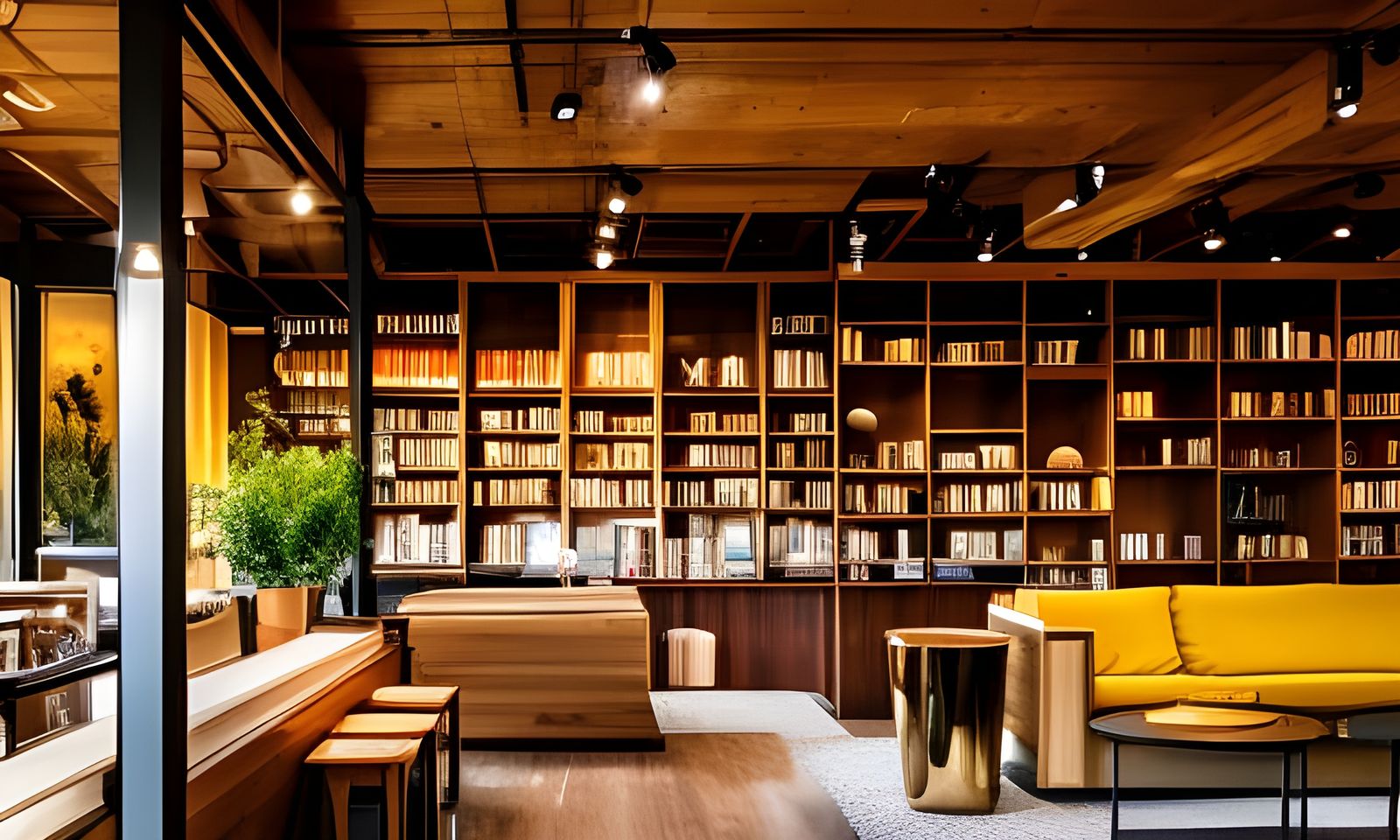The image depicts the interior of an upscale, hyper-realistic library, characterized by its luxurious use of mahogany wood. The ceiling and walls, adorned with deep mahogany, provide a rich, warm atmosphere. The back wall is lined with floor-to-ceiling bookcases, which are densely packed with hundreds of books featuring various spine colors including red, black, and white. The lower sections of these bookcases are solid, while the upper sections are open shelves, adding depth and visual interest.

In front of these bookcases, a bright taxi-yellow sofa with a light wooden base stands out vividly. The sofa is complemented by black wrought-iron coffee tables positioned in front of it. Adjacent to the sofa on the left side is a sizable brass garbage can that matches the sofa's height, adding a unique focal point. Further to the left, there's a wooden bar equipped with stools, suggesting a possible coffee bar area, accentuated by some black metal girders that extend up to the ceiling, creating a sense of structure and division within the space.

The room also includes additional seating and vertical dividers interspersed with greenery, bringing in bright green tones from the plants. The soft white lighting illuminates the room gently, enhancing the luxurious feel without being overly harsh. The warm brown and light brown wooden elements, the gray carpeting, and the vibrant yellow and green accents create a harmonious and inviting ambiance perfect for reading and relaxation.